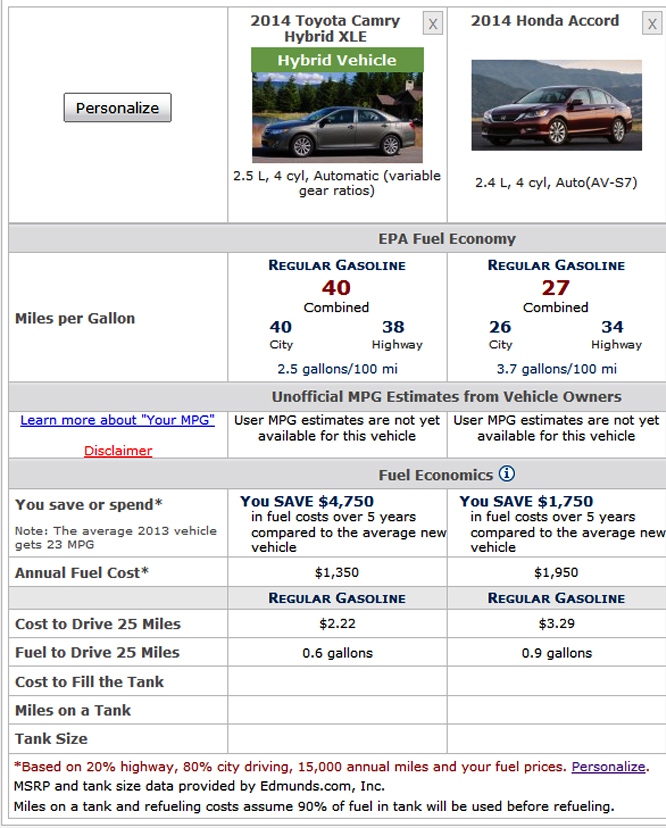The image features a light blue background with dark blue lines outlining the edges except on the right side, where it remains open. At the top of the image, a white box contains a smaller blue box with the word "Personalize" written inside. Below this, there are images and details of two different cars: 

1. **2014 Toyota Camry Hybrid XLE:**
   - There is a small box with an "X" in the top right corner.
   - A green box across the car's image indicates "Hybrid Vehicle."
   - The details about the vehicle include information on its cylinders and specifications.

2. **2014 Honda Accord:**
   - Similar to the Camry, it has a small box with an "X" in the corner and a description of the car’s features.

Below the vehicle descriptions, a detailed section on EPA fuel economy is displayed in a blue box, covering the following metrics:
- **Miles per Gallon (MPG) for Regular Gasoline:**
   - Combined: 40 MPG
   - City: 40 MPG
   - Highway: 38 MPG
   - Consumption: 2.5 gallons per 100 miles (for one set of data)
   - Combined: 27 MPG
   - City: 26 MPG 
   - Highway: 34 MPG
   - Consumption: 3.7 gallons per 100 miles (for another set of data)
- A blue box underneath reads "Unofficial MPG estimates from vehicle owners. Learn about your MPG," with "Learn about your MPG" in blue and underlined.
- A red underlined disclaimer states that "User MPG estimates are not yet available for this vehicle."

Further down, another blue box titled "Fuel Economics" includes a circle with an "i" inside it. This section elaborates on:
- Savings or additional expenses.
- Annual fuel cost.
- Cost to drive 25 miles.
- Fuel cost per trip and cost to fill the tank.
- Miles achievable on a full tank.
- Tank size.

Specific figures are provided:
- $222 for one and $329 for another (possibly representing different fuel types or driving conditions).
- 0.6 gallons and 0.9 gallons consumption.
- A red footnote indicates that these figures are based on 20% highway and 80% city driving, assuming 15,000 annual miles and current fuel prices.

The bottom part emphasizes "Personalize" (underscored) and notes that the MSRP and tank size data are provided by Edmunds.com Incorporated. It also mentions that refueling costs assume 90% of the tank will be used before refilling.